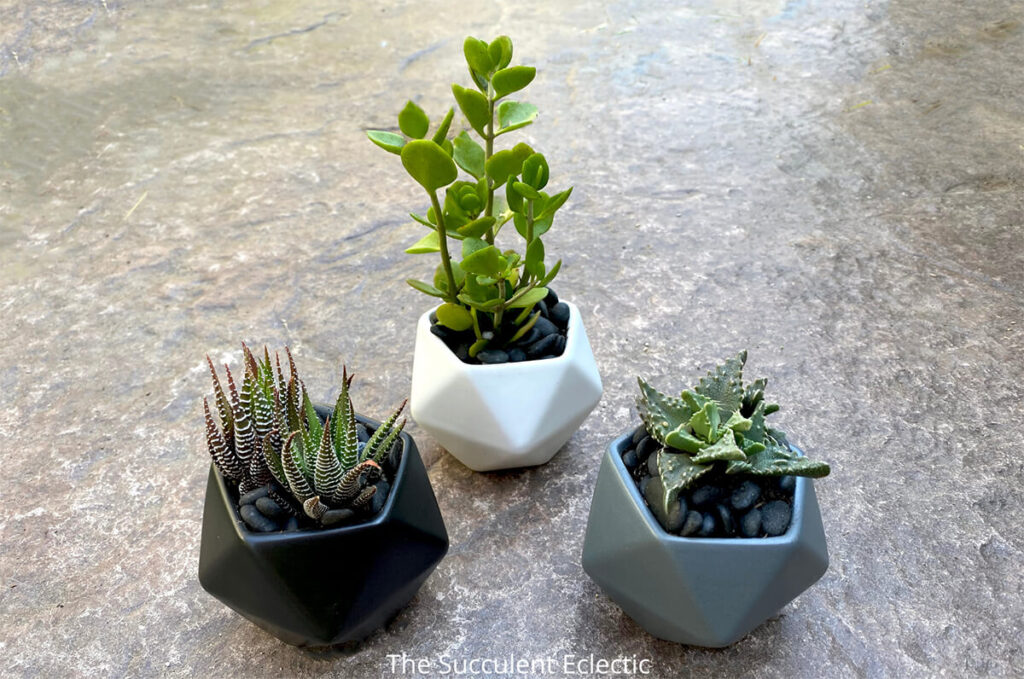The image showcases three distinct succulent plants, each housed in a uniquely colored geometric vase — one black, one white, and one chromic blue. The vases share a tessellated triangular pattern, forming a faceted, prism-like shape with pentagonal openings at the top. Each vase is filled with black pebbles, providing a stark contrast to the vibrant greenery of the plants. The plants appear to be different species of cacti or succulents: the black vase on the left contains short, spiky tendrils; the central white vase holds tall, vine-like stems with thick leaves; and the blue vase on the right features flat, triangular, ridged leaves. They are arranged on a gray, stone-like surface with a few ridges, giving a textured background to the composition. The clear photograph is finished with white text at the bottom center, reading "The Succulent Eclectic."